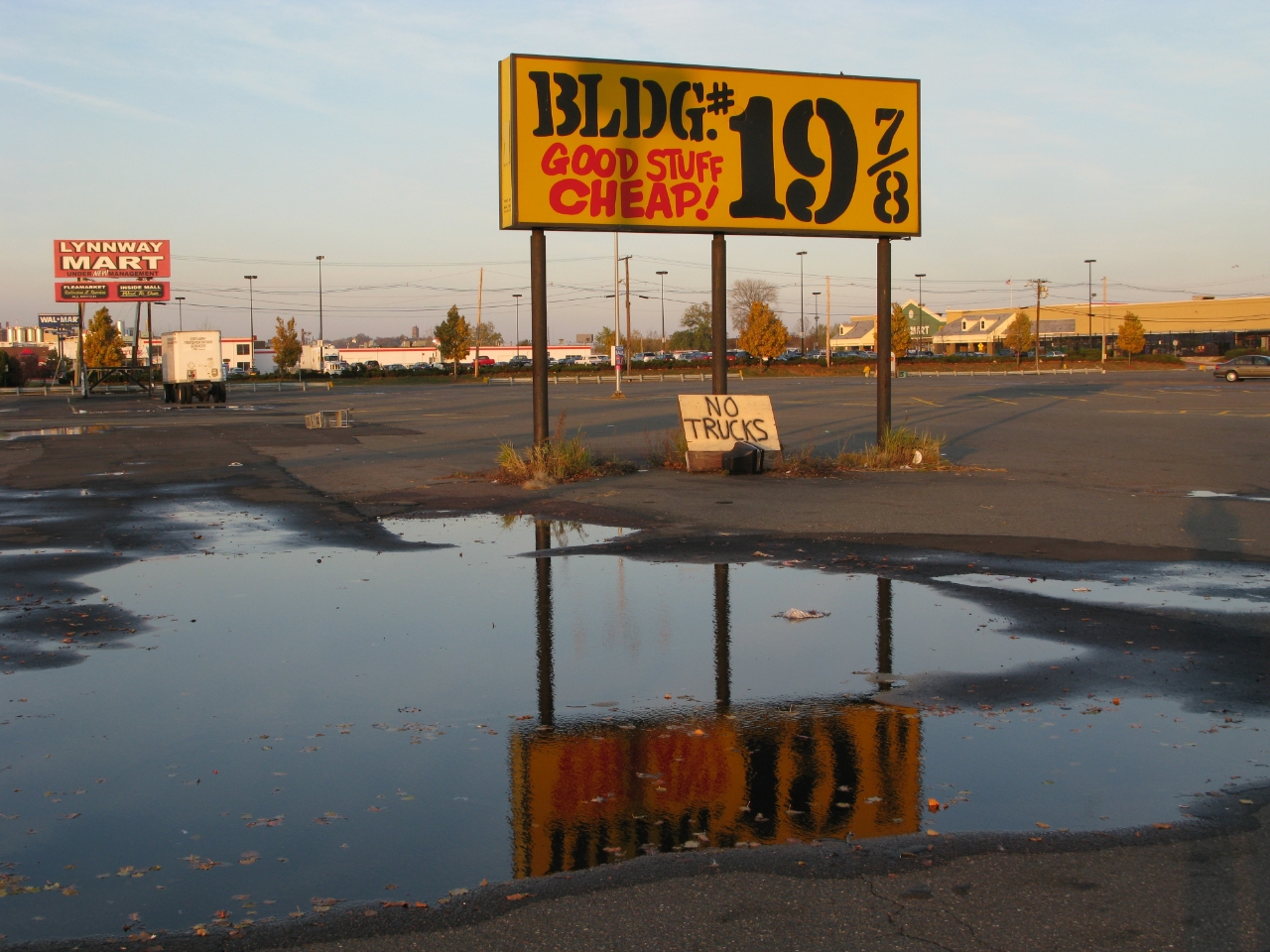In the early morning light, a deserted asphalt parking lot captures the serenity of dawn. The sun casts a gentle glow, revealing a vast empty space interrupted only by a large puddle of water in the foreground, reflecting the bright blue sky. Dominating the scene is a large rectangular sign, mounted on three sturdy metal poles. The sign prominently displays "Building Number 19-7-7-8" in bold black letters, and just below, "Good Stuff Cheap!" in striking red letters, hinting at the value within. Off to the right, at the far end of the parking lot, a strip mall comes into view. Its front entrance stands out with a distinctive blue canopy supported by stone or brick pillars. Beneath the large orange sign, a smaller, white sign leans against one of the pillars, bearing the simple message, "No Trucks." The combination of empty space, early sunlight, and clear signage paints a detailed picture of a quiet and inviting commercial area ready to welcome the day's visitors.